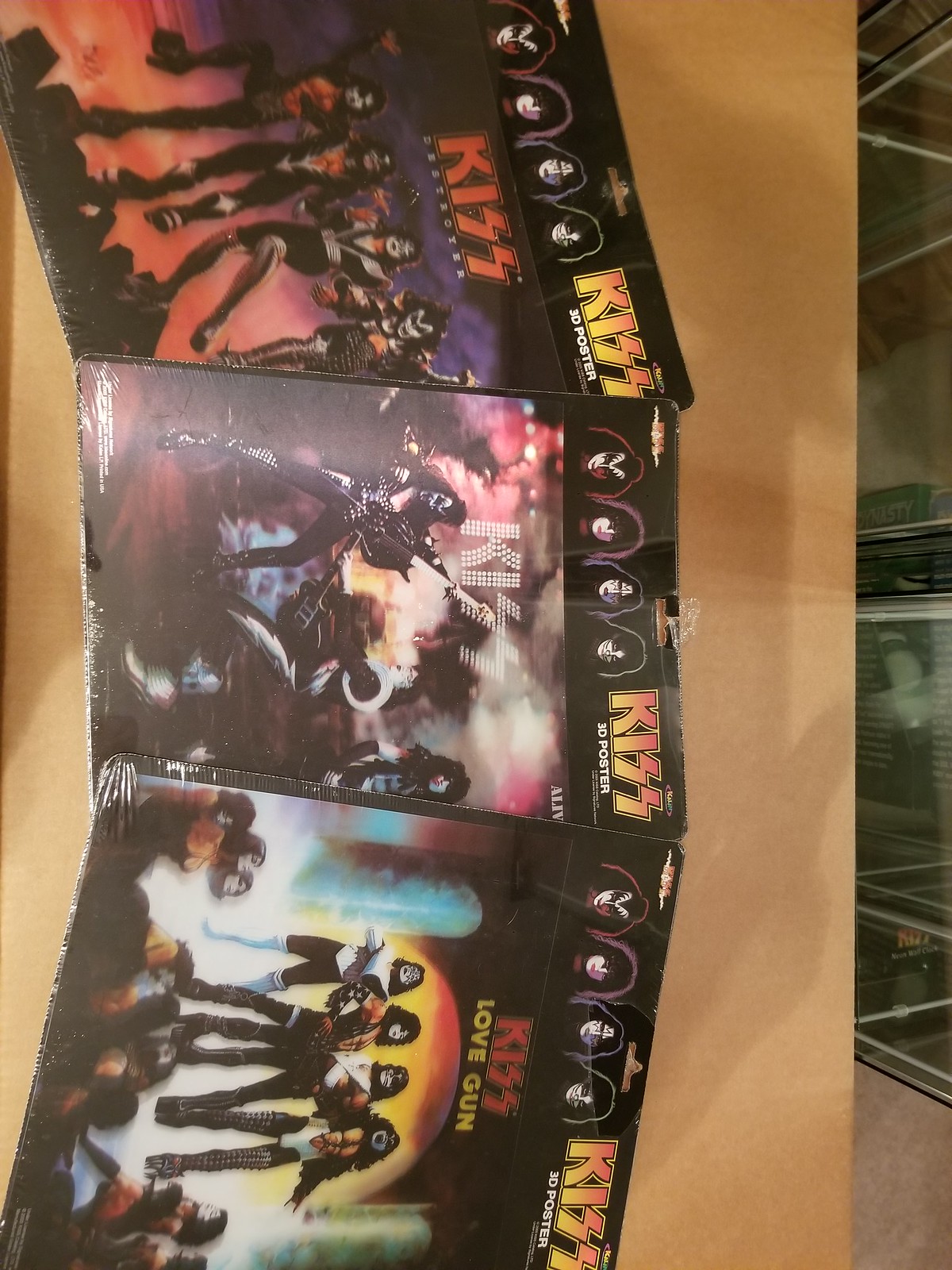The image depicts three 3D posters of the band KISS, oriented incorrectly, requiring a 90-degree anti-clockwise rotation to be viewed correctly. The photograph taken from an aerial perspective shows the posters placed on top of a light brown cardboard surface, with the posters slightly overlapping each other. The one on the far right partially rests on the middle poster, which in turn rests on the leftmost one. Each poster features a prominent KISS logo at the top, with variations in the color of the text—orange, yellow, red, white—with an additional "3D poster" label beneath. The posters exhibit images of the band members in their iconic makeup and costumes, engaged in activities like playing instruments or posing dramatically. Notable imagery includes a scene with the band performing in costume and a "Love Gun" themed poster with striking red and yellow fonts, depicting the band in a dramatic pose before an audience. The dark, black backgrounds of the posters contrast with the reflections and stretch marks visible on the plastic shrink wrap packaging, indicating the items are unopened. The shadows cast across the cardboard add depth to the composition, hinting at the ambient lighting conditions when the photograph was taken.